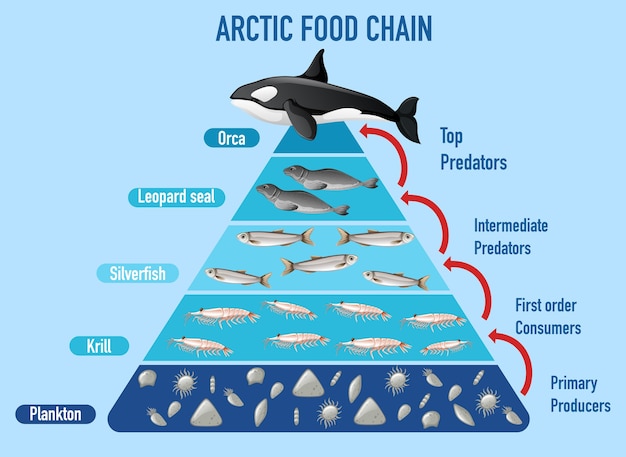This detailed illustration depicts the Arctic food chain organized as a pyramid against a medium cool blue background, with each level transitioning through various shades of blue. At the apex of the pyramid is an orca whale, labeled as the top predator. Directly beneath the orca are leopard seals, categorized as intermediate predators. Following the leopard seals are silverfish, which are designated as first-order consumers. Below the silverfish, krill are positioned as primary consumers. At the base of the pyramid, plankton are identified as primary producers. The diagram features red arrows indicating the flow of energy from the base to the top of the food chain, though the predominant color theme remains blue. The text "Arctic Food Chain" is prominently displayed in dark blue at the top, emphasizing the hierarchical structure of marine life in the Arctic ecosystem. This scientific diagram, possibly from an educational book or biology website, provides a clear visual representation of the interconnected relationships among Arctic marine species.